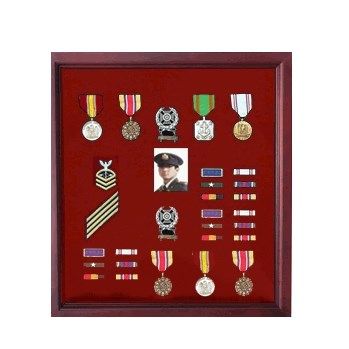The image showcases a meticulously arranged framed display of military medals and insignia set against a dark red velvet background. The frame itself is crafted from cherry wood with a white matting around the edges, enhancing the display. At the top of the frame are five distinct medals, including silver, bronze, and gold, accompanied by a striking Navy Cross and a marksmanship medal. Notably, above these medals are colorful ribbons: maroon and gold, light beige and pink, green, and white. 

Centrally placed in the frame is a small photograph of a soldier in uniform, wearing a hat that partially obscures their face. Surrounding the photograph are various badges, patches, and insignia that would typically be worn on a military uniform, including a U.S. Navy petty officer insignia on the left. At the bottom of the frame, three more medals are displayed, bringing the total count to seven, including another marksmanship medal. The entire composition appears to be an homage to a distinguished U.S. serviceman, reflecting their commendable service and participation in multiple campaigns.